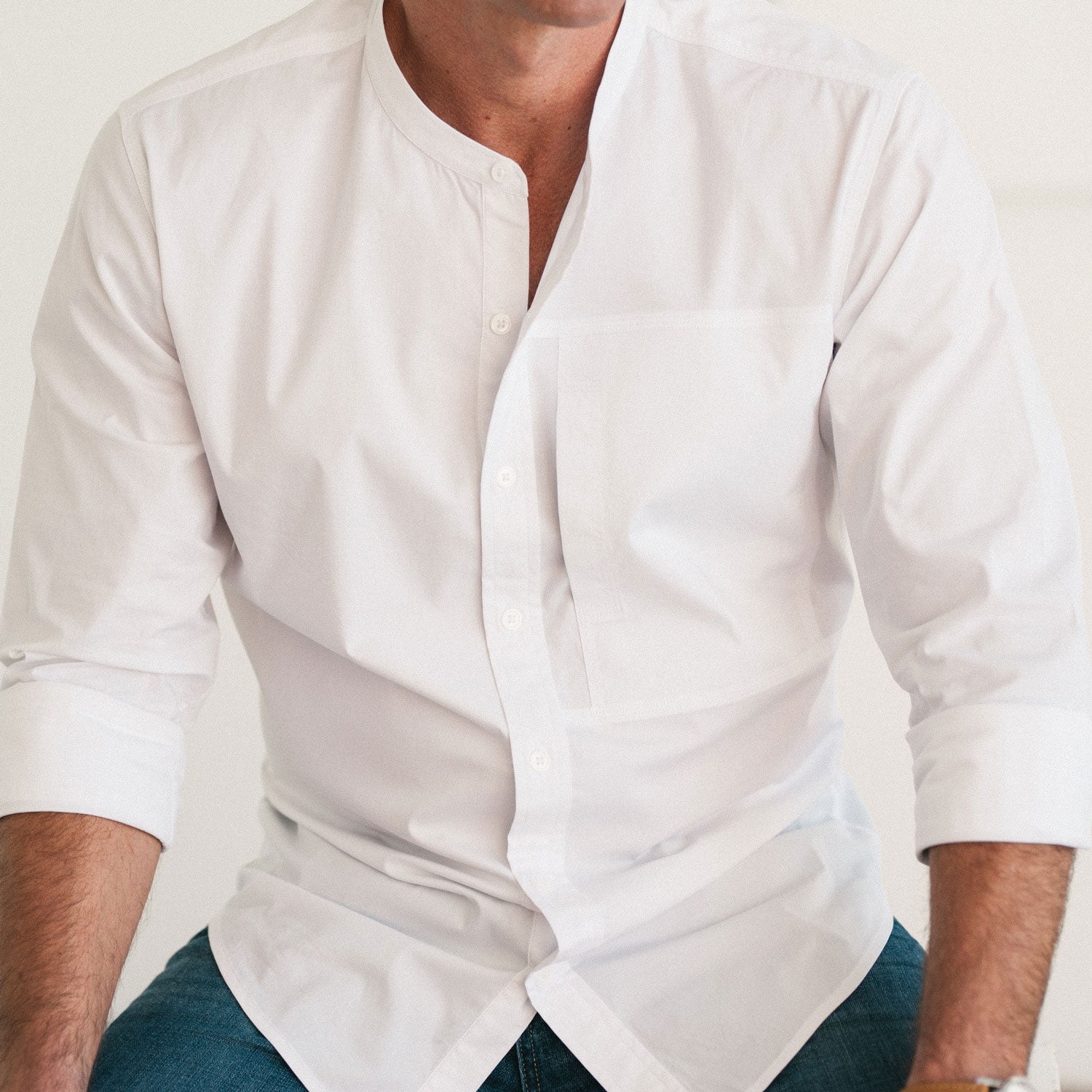The image depicts a male model, photographed from just below the tips of his chin down to his hips. He is dressed in a white long-sleeved dress shirt, with the top two buttons unbuttoned, revealing a hint of his muscular chest. The sleeves of the shirt are rolled up to reveal the bottom third of his arms, which are noticeably hairy and suggest the model is Caucasian. His prominent Adam’s apple is visible, adding to the defined and chiseled appearance. The man’s white shirt includes a pocket on the left side of his chest, and he is paired with blue denim jeans. The photograph has a professional feel, with a stark white background that accentuates the model's attire and physique. His hands are not visible, as they are positioned below the base of the image, likely resting on his lap. The overall look carries the semblance of an advertisement, highlighting the model's partial yet distinct, fashionable style.